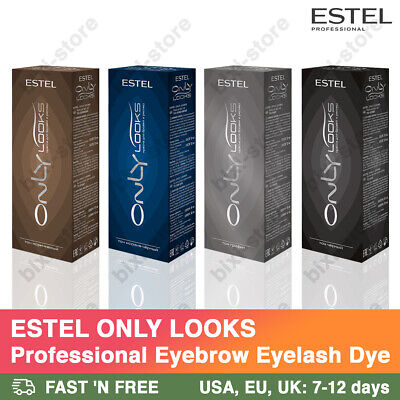The image showcases a collection of four product boxes neatly displayed above a promotional banner. The top portion of the banner is orange, transitioning into a thinner green line at the bottom, with white text that reads, "Estelle, E-S-T-E-L, Only Looks Professional Eyebrow Eyelash Dye." A small graphic of a truck accompanies text indicating a fast and free shipping offer to the USA, EU, and UK, with an estimated delivery time of 7-12 days.

The four boxes on display are each of a different color: brown, blue, gray, and black. At the center of each box, "Only Looks" is prominently printed in white font. Near the top of the boxes, the brand name "Estelle" appears, with additional smaller print on the visible side of each box, though the text is not legible. In the upper right corner of the image, "Estelle Professional" is displayed with "Estelle" in larger black font and "Professional" in a smaller black font beneath it.